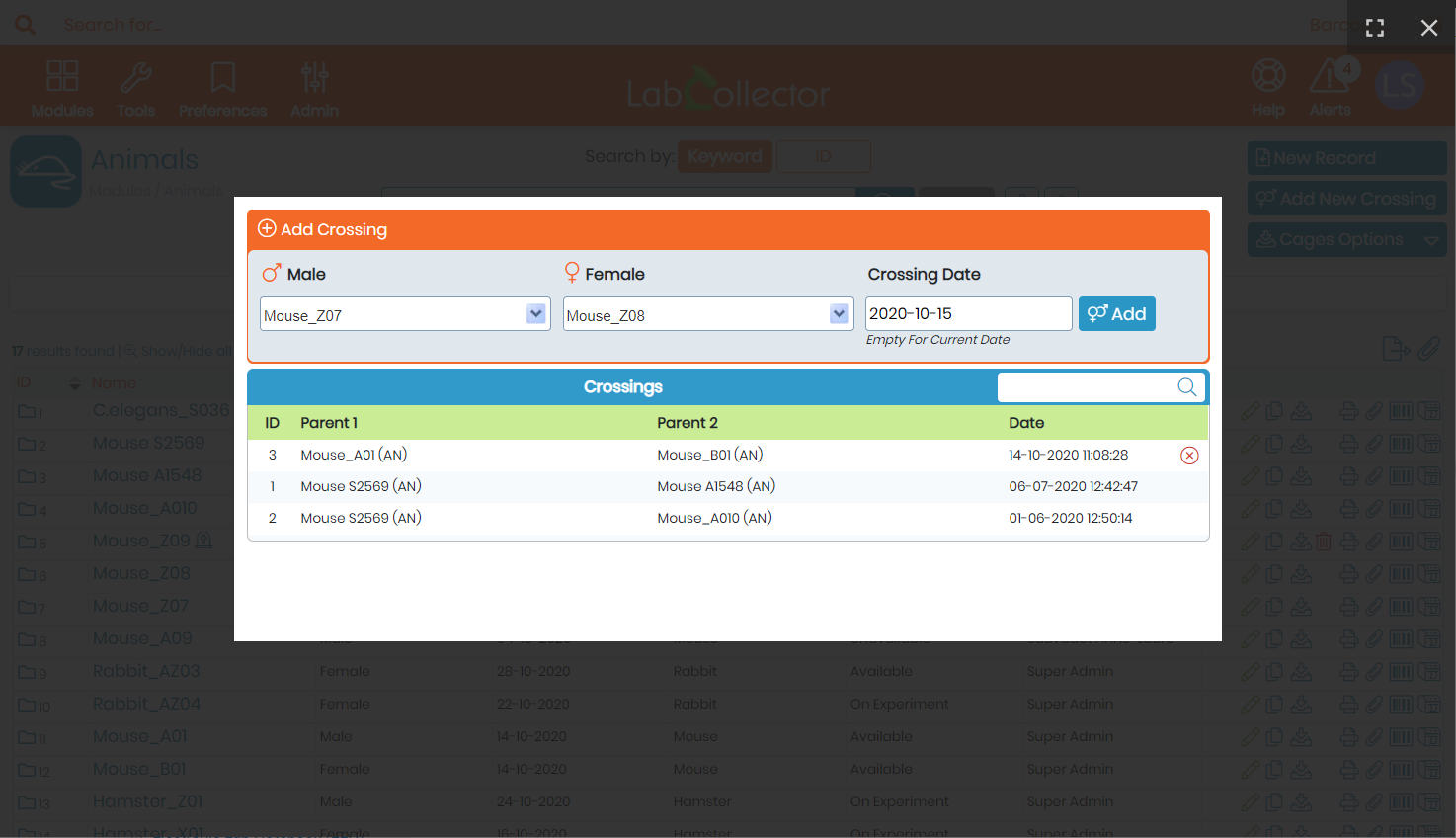The image depicts a computer screen displaying a laboratory data management interface. In the background, there is a main window showcasing multiple fields, each filled with textual information organized within boxes. Notably, in the top-right corner of the main window are buttons labeled "Help" and "Alert", while the top left features an assortment of icons. The focal point of the image, however, is a prominent pop-up window.

This pop-up window is distinguished by an orange bar at the top, which includes white text on the left that reads "Add Crossing" next to a plus symbol. Beneath this heading, there are symbols for male and female, each followed by the respective gender written in black. To the right of these labels is a section titled "Crossing Date," which displays a specific date: "2020-10-15."

Further details include identifiers for the mouse specimens involved: "mouse_707" for the male and "mouse_708" for the female. Below this information, there is a blue bar titled "Crossings" in white text, accompanied by a search box on the right. Within this section, there are rows labeled "ID 3," "1," and "2," followed by columns specifying "Parent 1," "Parent 2," and corresponding dates. Additionally, an 'X' icon is visible on the top right corner of the pop-up window, likely for closing or clearing the date entry.